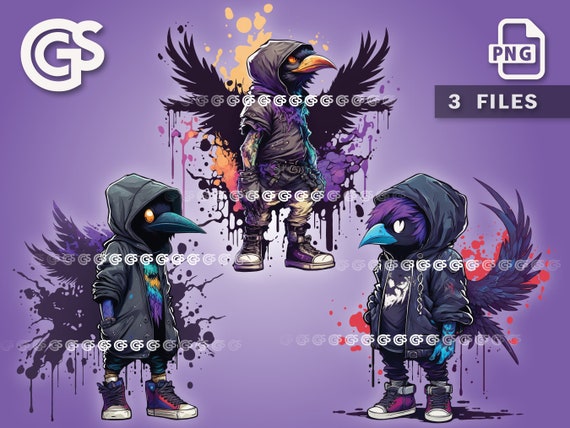This computer-generated illustration features three anthropomorphized bird characters set against a purple background. The upper left corner displays the initials "CGS" in white, while the upper right corner includes a white rectangle labeled "PNG" and the text "Three Files" underneath. The composition includes three crow-like figures, each standing upright and dressed in urban, gothic-style clothing that includes black hoodies, baggy pants, and high-top sneakers.

The central bird character is positioned slightly higher and sports a brown leather hoodie, beige pants, and dark purple high-tops. This bird has a striking golden beak and black wings extending from its back. To the left, the second bird wears a green hoodie with sleeves pushed up, revealing a vibrant pattern of teal, gold, blue, and purple feathers underneath. This character features a dark teal beak and yellow eyes, complementing its black high-top sneakers. The third bird on the right is adorned with a black windbreaker, showcasing distinct purple features, including a tuft of fur on its head, light blue beak, and blue hands. This bird's high-tops have notable purple accents, and it possesses a prominent purple tail.

Subtle details like the birds' colored eyes (ranging from yellow to white), the variety of their beak colors (from dark blue to light blue and yellow), and their dynamic postures add depth and character to the illustration. The entire scene is punctuated with colorful paint splatters in shades of yellow, purple, and red, adding an artistic flair to the detailed, edgy depiction of these humanoid birds.